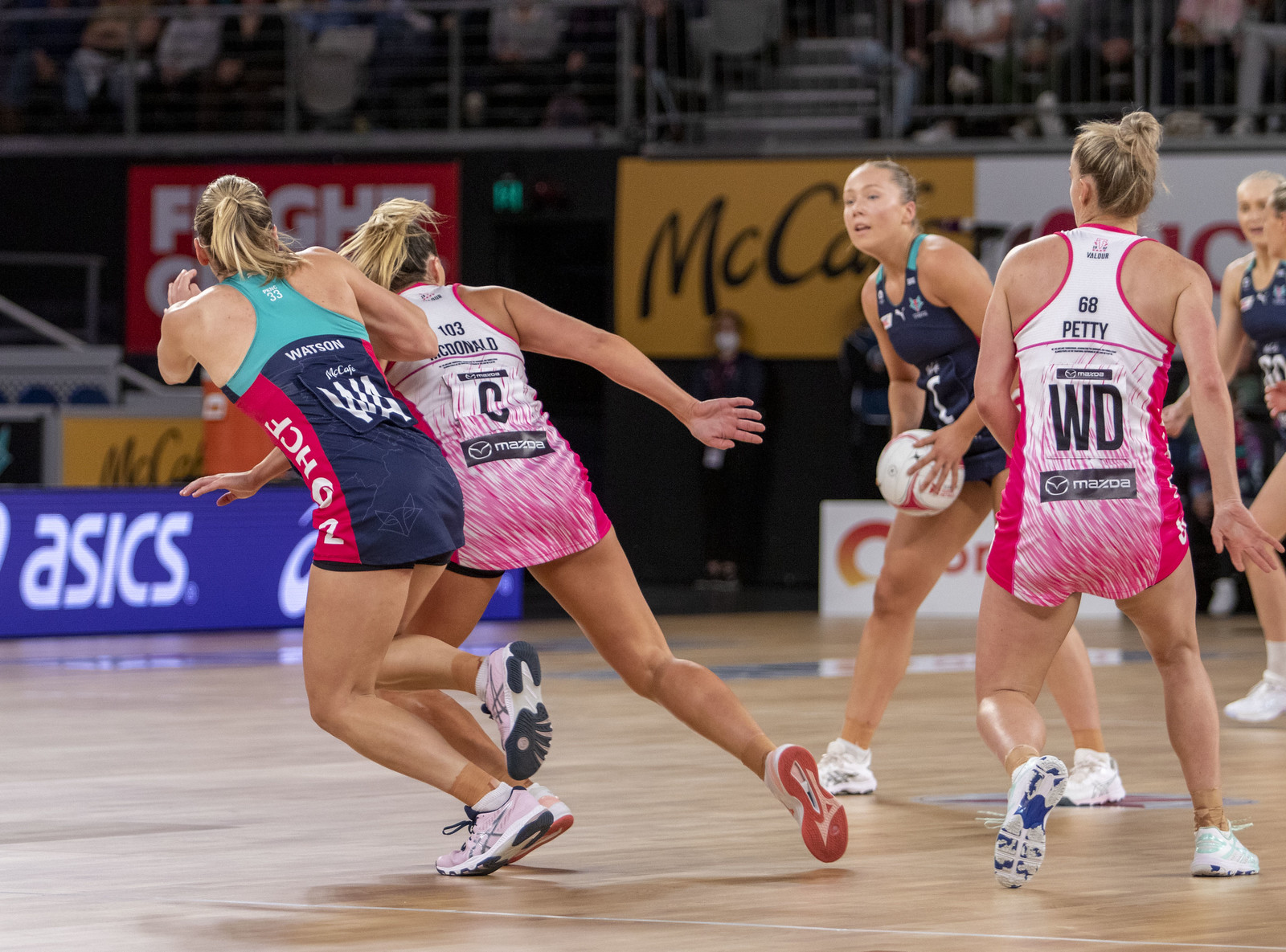This horizontal rectangular image, taken during an indoor women's basketball game, captures an intense action shot. A player in a red and white uniform holds the ball near her waist, preparing to pass it while scanning for an open teammate. She stands in the center of the image. To her right, her teammate, also in red and white, is positioned, while a player from the opposing team, dressed in an aqua-colored tank top with navy blue shorts and a red stripe, guards closely. The red and white jersey of one player prominently displays the number 103 and sponsors including McDonald and Mazda, while her teammate's jersey reads 68 with similar sponsorships. 

In the background, the stands are filled with blurred spectators and numerous advertisements, including visible logos and letters such as "ASICS" and "MCC." Few details can be deciphered, but one word, "fight," stands out in white. The scene is set on a polished hardwood floor, emphasizing the athletic intensity and fast pace of the game.